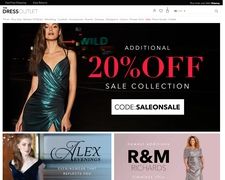The image primarily features a promotional advertisement with multiple elements. At the top left corner, there's the text "address outlet" accompanied by several icons aligned to the right. The header, which runs across the top of the page, is black. Directly below this, a black box displays a prominent "20% OFF" in large red letters, followed by the phrase "SALE COLLECTION" in uppercase gray letters beneath it. Below this, a white box contains the promotional code "SELL-ON-SALE".

On the left side of the advertisement, there is a woman wearing a dark green dress; her dark brown hair falls past her shoulders. Below this main section, there are two smaller advertisements. The one on the left features a different woman dressed in a black dress with the text "Alex Evenings" written beside her, although additional smaller text is unreadable. The smaller ad on the right has a pink background with the large bold letters "R&M".